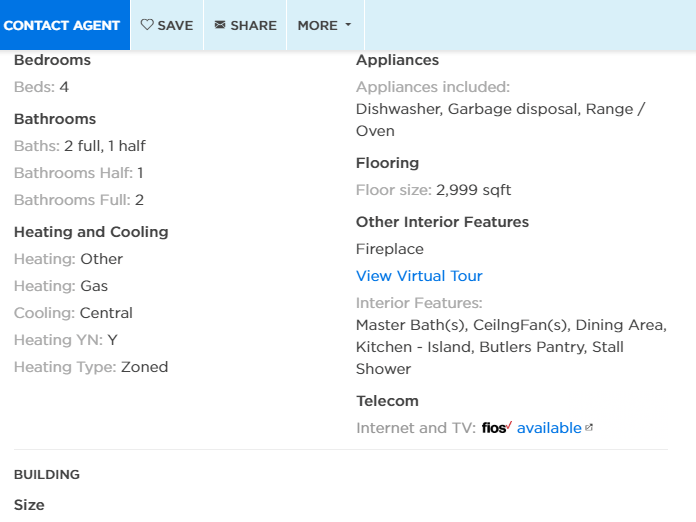This screenshot is a detailed listing of a house for sale or rent. At the top, a blue menu bar features an option labeled "Contact Agent," highlighted in darker blue. Below, a light blue bar with grey text contains the options "Save," "Share," and "More," with an arrow indicating additional clickable options. 

The left-hand side of the listing provides the home's specifications in bold and regular font. The property boasts 4 bedrooms ("Beds: 4") and 2 full bathrooms along with 1 half bathroom ("Baths: 2 Full, 1 Half"), further detailed as "Bathrooms: Half 1, Full 2." 

Under the "Heating and Cooling" section, the amenities include: "Heating: Other, Gas," "Cooling: Central," with tags "Heating YN: Y" and "Heating Type: Zoned." 

The appliances listed on the right include a dishwasher, garbage disposal, range, and oven. The home spans a "Floor Size: 2,999 Square Feet." Additional interior features include a fireplace.

A virtual tour, highlighted in blue, indicates various interior features such as a master bath, ceiling fans, dining area, kitchen island, butler's pantry, stall shower, telecom, and available internet and TV services.

The listing ends with a section titled "Building and Size," though details here are cut off in the screenshot.